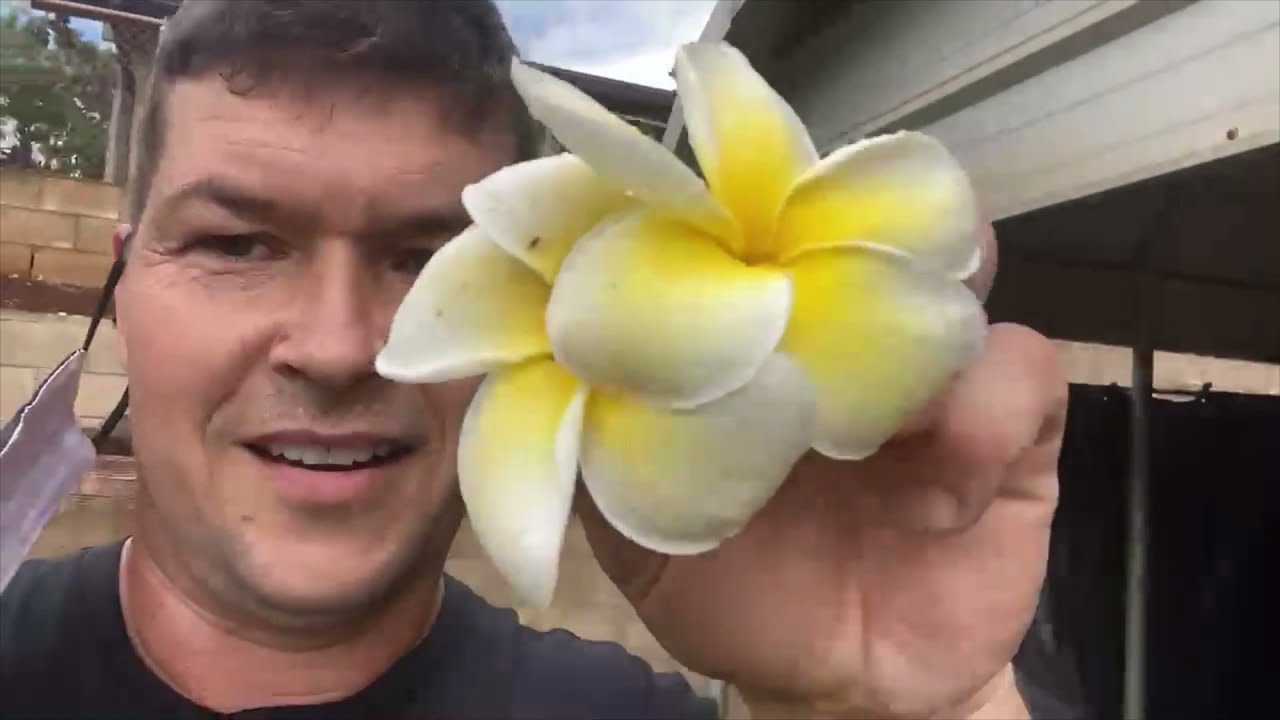In the close-up image, a Caucasian man with short brown hair, wearing a blue shirt, holds a large white and yellow flower in his left hand, raised next to his face. The flower is almost the size of his hand and has nine distinct petals with yellow towards the interior and white at the edges. The man’s face is partially obscured by the flower, revealing one full eye, part of his other eye, and his slightly ajar mouth showing his teeth. He appears to be staring directly at the camera with a hint of a smile, and a coronavirus mask hangs off his right ear. Behind him, the background includes a mix of bricks, a garage-like structure, some trees, a bit of blue sky with clouds, a cement wall, and a railing, placing him possibly in a suburban or residential setting.